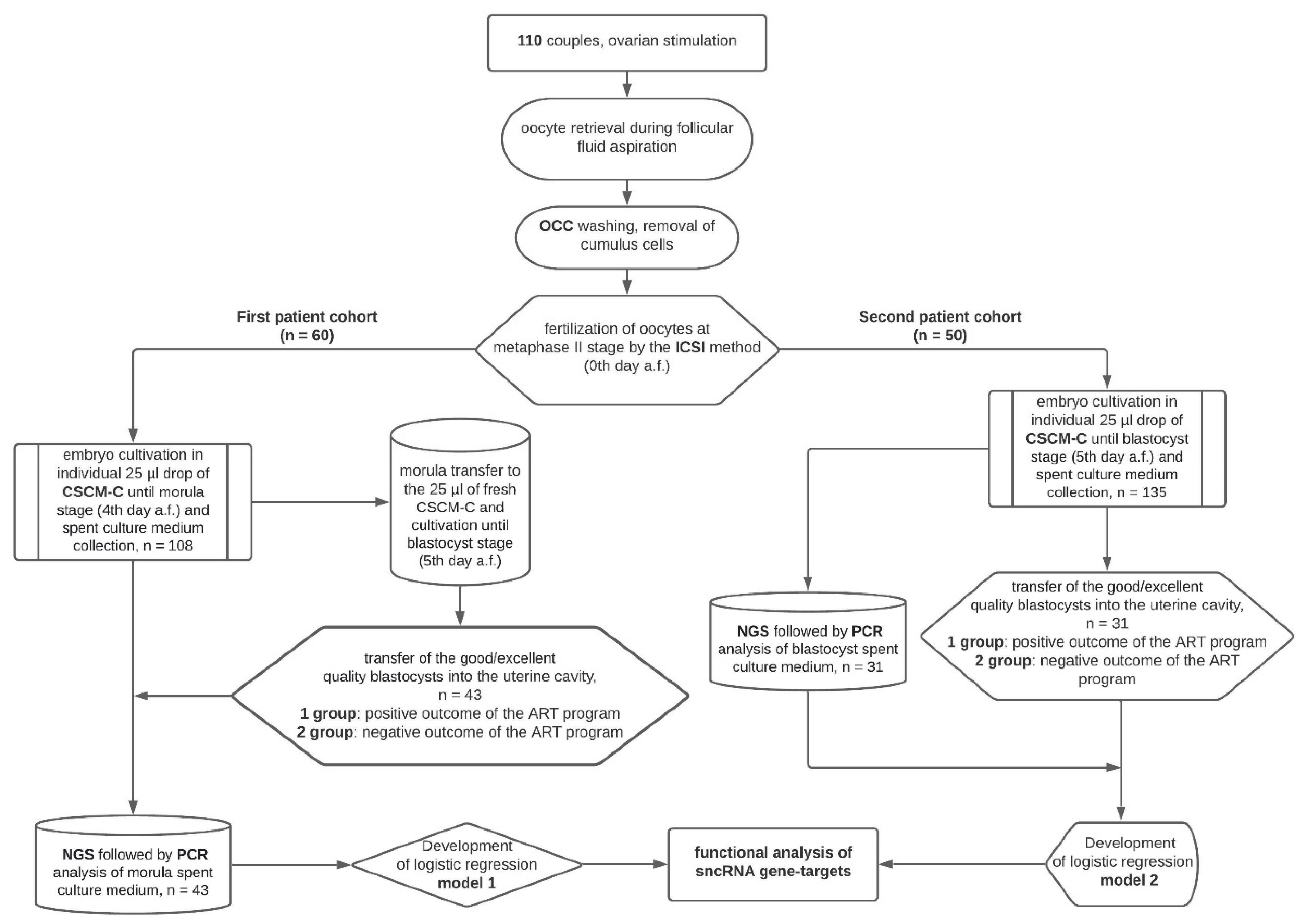The image is a detailed, black-and-white flowchart related to the fertilization of eggs in women. At the top of the diagram, it states "110 couples, ovarian stimulation," followed by steps including "oocyte retrieval during follicular fluid aspiration," "OCC washing," and "removal of cumulus cells." The diagram then branches into a larger section with black arrows connecting various shapes like ovals, rectangles, cylinders, and diamonds, each containing detailed descriptions of different stages and processes. Notably, the chart includes two distinct cohorts: the left section labeled "first patient cohort (N=60)" and the right section labeled "second patient cohort (N=50)." Further down, the diagram touches upon "fertilization of oocytes" and "metaphase," leading to the "development of logistic regression model 2" and mentions about "RNA gene targets." The overall setting is bright and clear, with each section of the flowchart providing detailed information, contributing to the complexity of this reproductive experiment.